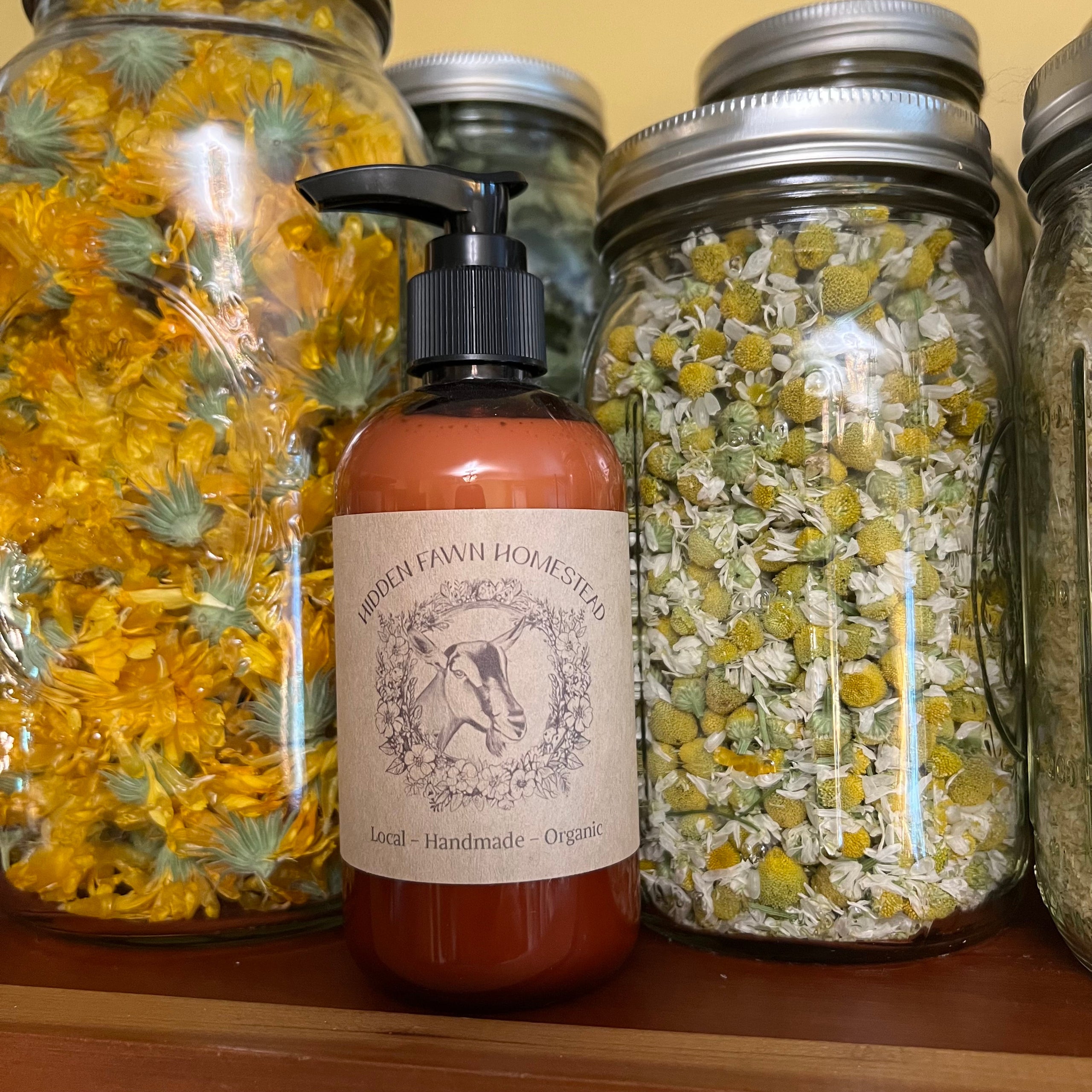In this detailed photograph, a handmade product is prominently featured on a wooden shelf. At the center is a reddish plastic pump bottle, potentially containing lotion or soap. The bottle is capped with a black pump dispenser and partially filled with a brown liquid substance. The rustic label adorning the front features an illustration of a goat's head encircled by a floral wreath, with "Hidden Fawn Homestead" inscribed above and "Local Handmade Organic" at the bottom. Nestled around the central bottle are glass mason jars filled with assorted flowers – the jar to the right brimming with a profusion of small daisies, while the jar to the left holds an array of yellow blossoms, reminiscent of dandelions. This arrangement beautifully highlights the artisanal quality of the product on display.